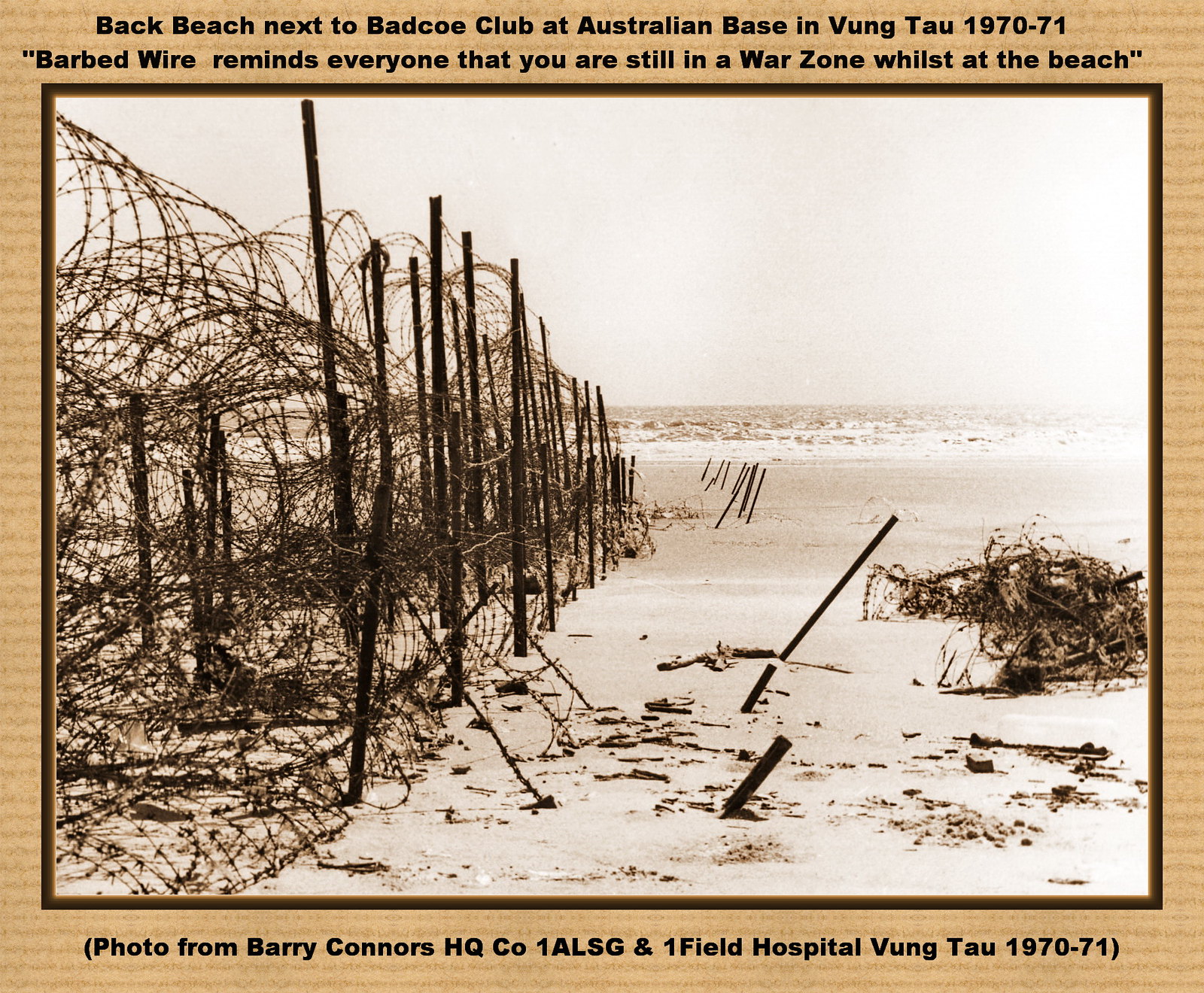This sepia-toned photograph, bordered by a matte tan paper frame adorned with black text, vividly captures a wartime beach scene. The text at the top reads, "Back Beach next to Bad Co. Club at Australian Base in Vung Tau, 1970-71," and a reminder in the middle underscores, "Barbed wire reminds everyone that you are still in a war zone whilst at the beach." At the bottom, the photo is credited as, "Photo from Barry Connor's HQ CO 1 ALSG and One Field Hospital, Vung Tau 1970-71." Central to the image is a beach, visually anchored by barbed wire stretching across the left, held up by tall metal poles. This foreboding fence contrasts sharply with the serene ocean glimpsed in the distance and the expansive sky above. Scattered poles and possibly a pile of twisted barbed wire or seaweed hint at the chaotic presence of military infrastructure amidst the natural setting. Although devoid of people, the image powerfully juxtaposes the inherent beauty of the beach with the harsh reminders of the ongoing conflict in Vietnam during the time it was taken.